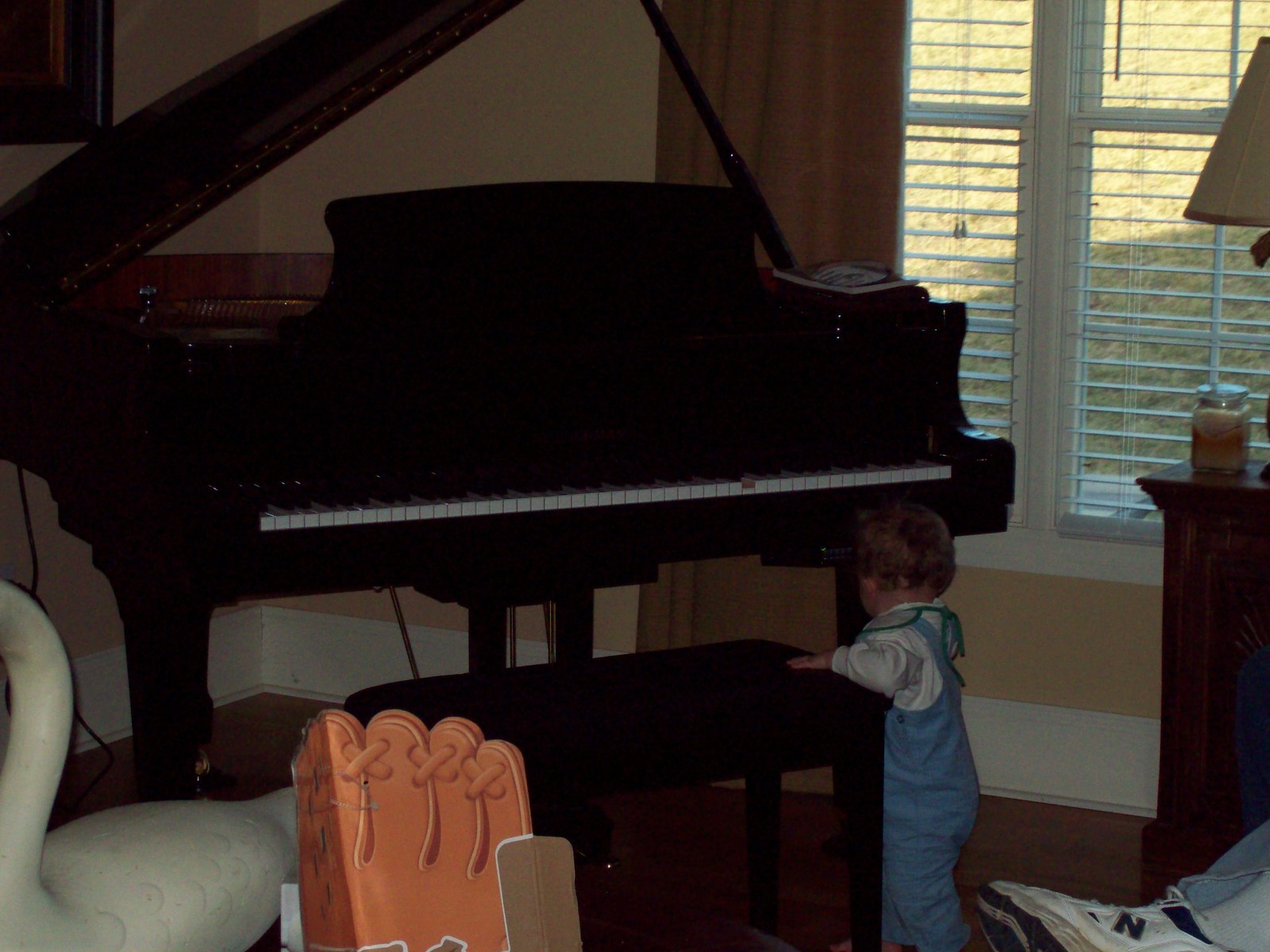In an intimate living room setting with wooden flooring and light pouring in from a window partially covered by floor-length brown curtains, the centerpiece is a sleek black baby grand piano with its lid propped open by a black stick. Positioned directly in front of the piano is a matching bench, and leaning against it is a toddler with brown hair dressed in blue overalls and a white shirt, his back to the viewer. The corner of a table with a cream-colored lampshade atop a lamp and an unlit candle is visible near the window. Amidst the backdrop of cream walls, the scene on the left showcases a cardboard cutout of a baseball glove and a swan statue, while on the right, the edge of the picture reveals a white tennis shoe with an "N" on it, partially obstructed by jeans. The diverse color palette features black, white, brown, tan, green, gray, light blue, and orange, capturing a serene midday indoor atmosphere.